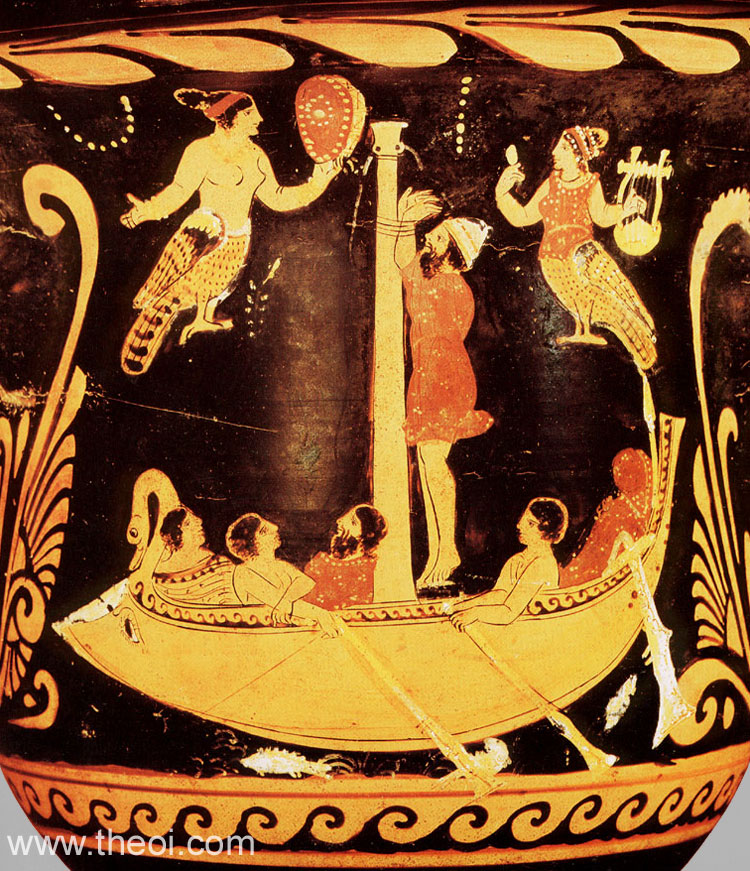This image depicts a detailed and stylistic scene reminiscent of ancient Grecian artwork on what could be a vase, urn, or cup with a matte black background and a decorative pale yellow and red design. In the lower section, there is a boat with a swan or duck-shaped bow. The boat contains four or five figures, some adorned in red clothing, one of whom is tied to a central mast. This individual, possibly a man, is being tormented by harpies—mythical creatures with women's upper bodies and birds' lower bodies. One harpy, positioned to the left and topless, holds a piece of meat or food, while her counterpart on the right wields a harp. Above the scene, there are yellowish-tan ornamental leaves wrapping around the top edge, accompanied by decorative gold symbols on both sides. The bottom border features a gold trim with a thin red line and black wave patterns, framing the entire composition.